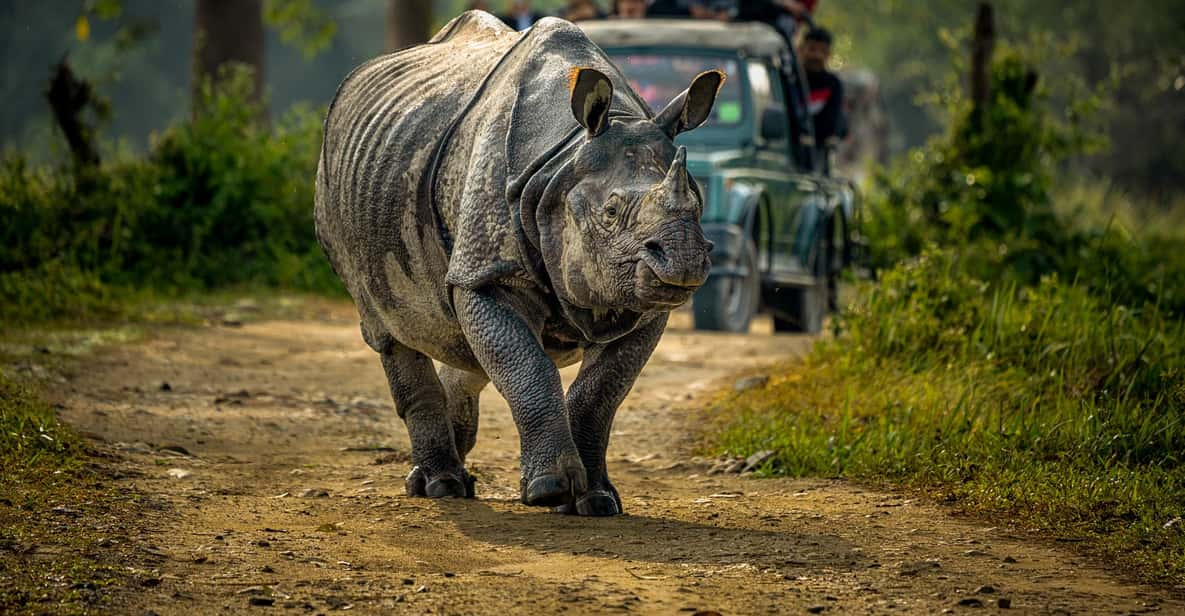In this clear and detailed photograph, an Indian rhinoceros with a short horn and a wrinkly hide, dotted with patches of dried mud, stands on a dirt road, staring directly at the camera. The road is flanked by lush green grass and dense trees, which blur slightly at the upper corners of the image, adding a dreamy quality to the scene. Behind the rhinoceros, there's a blue-green Jeep truck teeming with Indian spectators, some standing and others holding up phones to record the encounter. It appears to be a safari vehicle possibly overfilled with eager onlookers hoping the rhinoceros will move so they can proceed. The scene suggests a rich, immersive safari experience in a forested area.